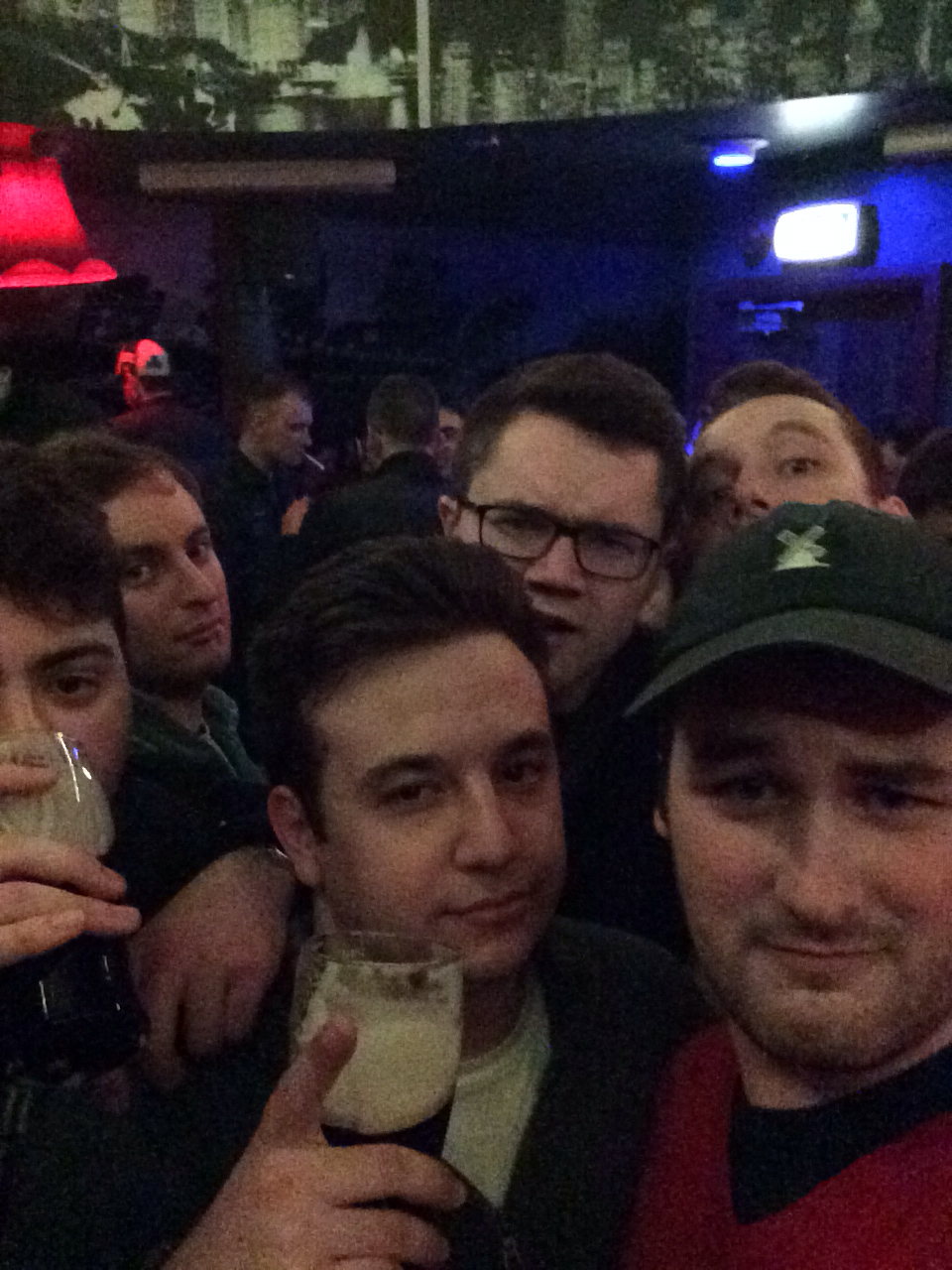This photographic image captures a close-up scene inside a dimly-lit bar, featuring a group of Caucasian men, all looking toward the camera. In the bottom right-hand corner, a man with a gruff stubble and dark eyes is slightly smiling. He wears a gray hat adorned with a windmill emblem and a red and black shirt. His left arm is draped around the shoulder of the man next to him, who is holding a beer glass mostly filled with foam. This man, sporting a white shirt under a dark jacket, has dark hair and dark eyes and is pointing his index finger upward.

To his left, a man with his hand on the shoulder of the beer-holding man is captured in the act of lifting his own glass of dark beer, seemingly preparing to drink it. His glass is held aloft, close to his face. Behind this central trio, another man with glasses, dark hair, and dark eyes peers directly into the camera. Further to the left, another man inclines his head slightly, also looking straight at the camera without smiling.

In the background, partially obscured, is another man wearing a hat, his face turned upwards as he tries to catch sight of the camera. The ambiance includes elements of a bustling bar scene: a white man smoking a cigarette, red lights or lampshades, and what appears to be a spotlight. No text is visible in the image, drawing complete focus to the detailed expressions and interactions of the men within this intimate bar setting.